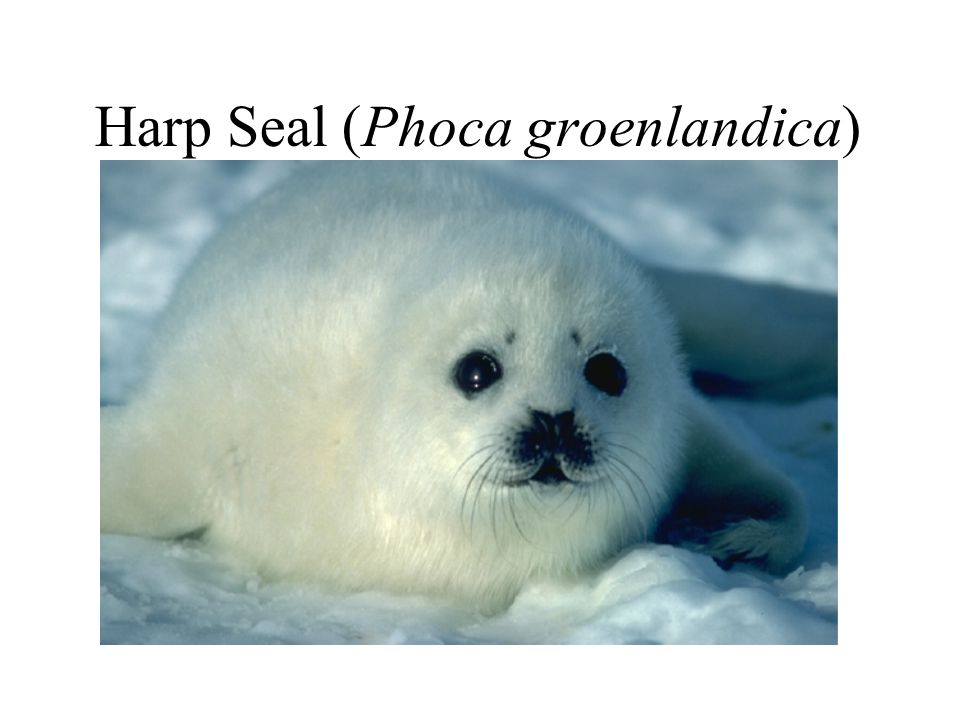The image depicts a young harp seal (Harp Seal, Phocogroenlandica) resting on snow outdoors. The seal, which is white in color, has glimmering fur and distinct black features: beady eyes, a small nose, whiskers, and minute dot-like eyebrows. The seal gives an impression of contentment as it lies on a bluish-gray snow bed, with the shadow on its right suggesting the sun's presence. The image is clear, with text at the top in black displaying "Harp Seal" and "Phocogroenlandica" in parentheses, indicating the seal's common and scientific names.